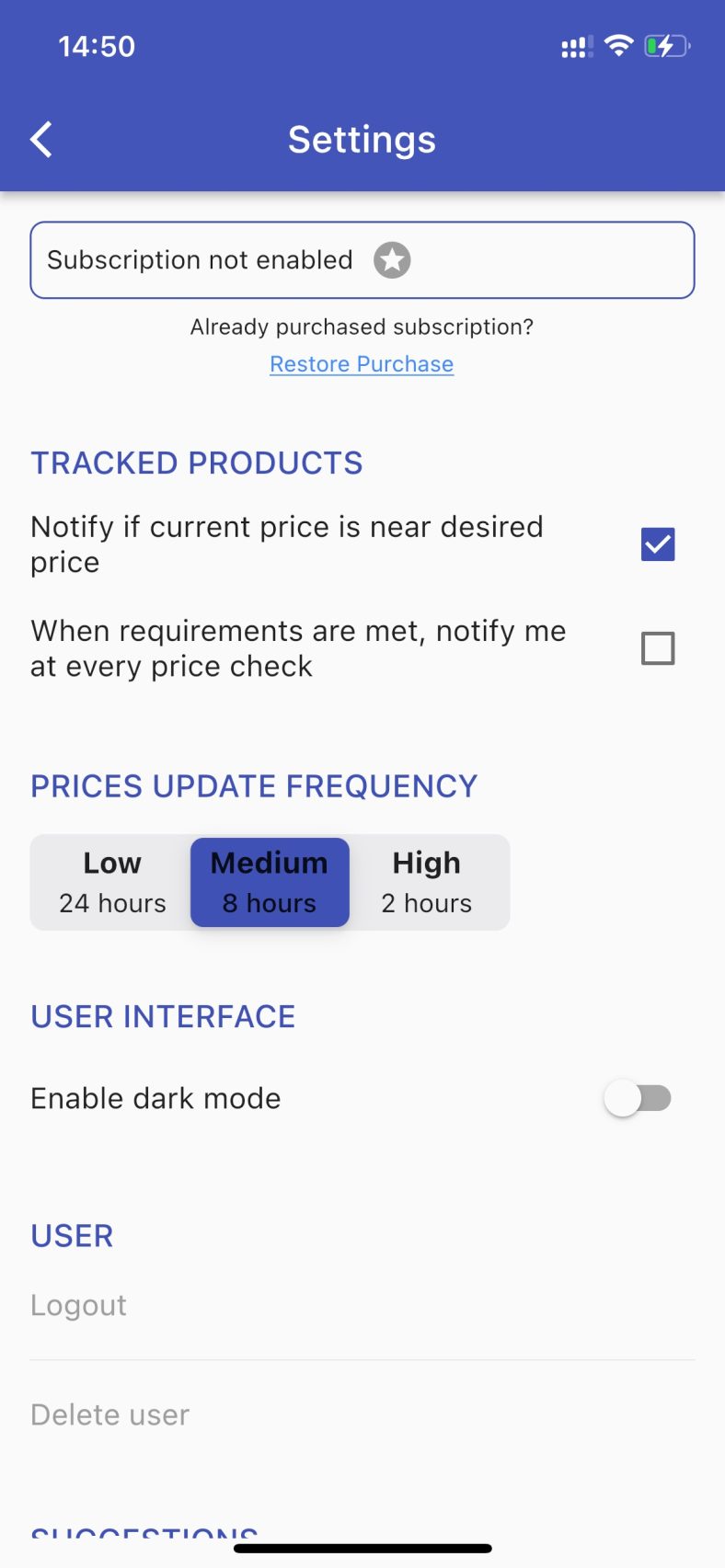This screenshot captures a detailed interface of a price drop alert app for Android phones. The top header is adorned in periwinkle, prominently displaying the title "Settings." Beneath the header, the body of the app is showcased with a clean white background. A notification bubble at the forefront alerts the user with the message "Subscription not enabled," accompanied by a grey star symbol.

The first section on the page, titled "Tracked Products," lists two options:
1. "Notify if current price is near desired price" – marked by a checked checkbox indicating activation.
2. "When requirements are met only notify me at every price check" – paired with an unchecked, blank checkbox.

The second section, "Prices Update Frequency," offers a choice of three intervals, each represented by a bubble:
- Low: 24 hours
- Medium: 8 hours, highlighted in periwinkle to indicate selection
- High: 2 hours

Moving to the third section, "User Interface," the option to enable dark mode is visible but currently not toggled.

The final section, "User," lists two options – "Log out" and "Delete user" – both of which are displayed in a grayed-out state, suggesting they are currently inactive.

Overall, the clear and organized layout presents a comprehensive view of the app's settings page, detailing various customizable features for the user's convenience.